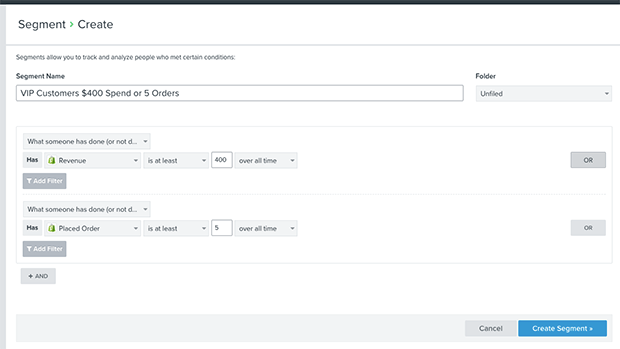The image displays a segment creation interface for a Shopify store. The background is mostly white, and the text appears slightly blurred. At the top, the header states, "Segment allows you to track and analyze people who meet certain conditions."

Below the header, there's a section titled "Segment name" with an input field labeled "VIP customers: $400 spent or five orders." To the right of this field, there's an indication of the folder being unspecified with the label "Folder: Untitled." Underneath the segment name section, it explains, "What someone has done or not done."

Several conditions for the segment are listed:
1. "Has revenue, is at least $400, over all time," with an option to add another filter.
2. A second condition mirrors the first but specifies "five orders," indicative of the criteria set by the segment's name.

On the bottom right of the interface, there are two buttons— "Cancel" and "Create Segment," with the latter highlighted in blue to proceed with the segment creation.

These options allow the Shopify store owner to categorize and manage VIP customers who either spent at least $400 or placed five orders, enhancing targeted analysis and engagement.